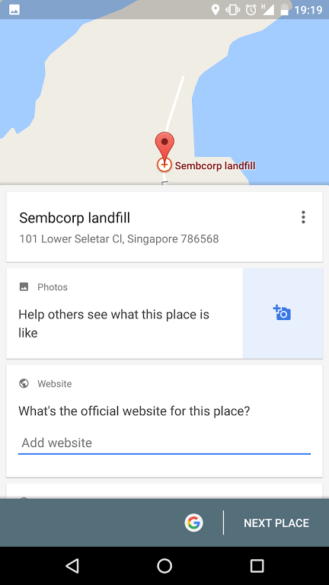Screenshot of a mobile device displaying a map with various icons. The top part of the screen shows the standard mobile interface, including symbols for battery level, the time (19:19), location services, an alarm, and Wi-Fi signal strength. 

Beneath this, the screen is partially covered by a map with an illustrated background. The background features water regions on both the left and right sides, while the land occupies the center. A red symbol marks a specific location on the land, identified as "Sembcorp Landfill."

Further down, overlaying the map background, there are several white banners. The first white banner contains black text detailing the location: "Sembcorp Landfill," followed by the address "101 Lower Seletar, Singapore 786568."

The next banner encourages user interaction, stating: "Photos help others see what this place is like." Below this, another prompt invites users to add the official website for this location, stating: "Add website."